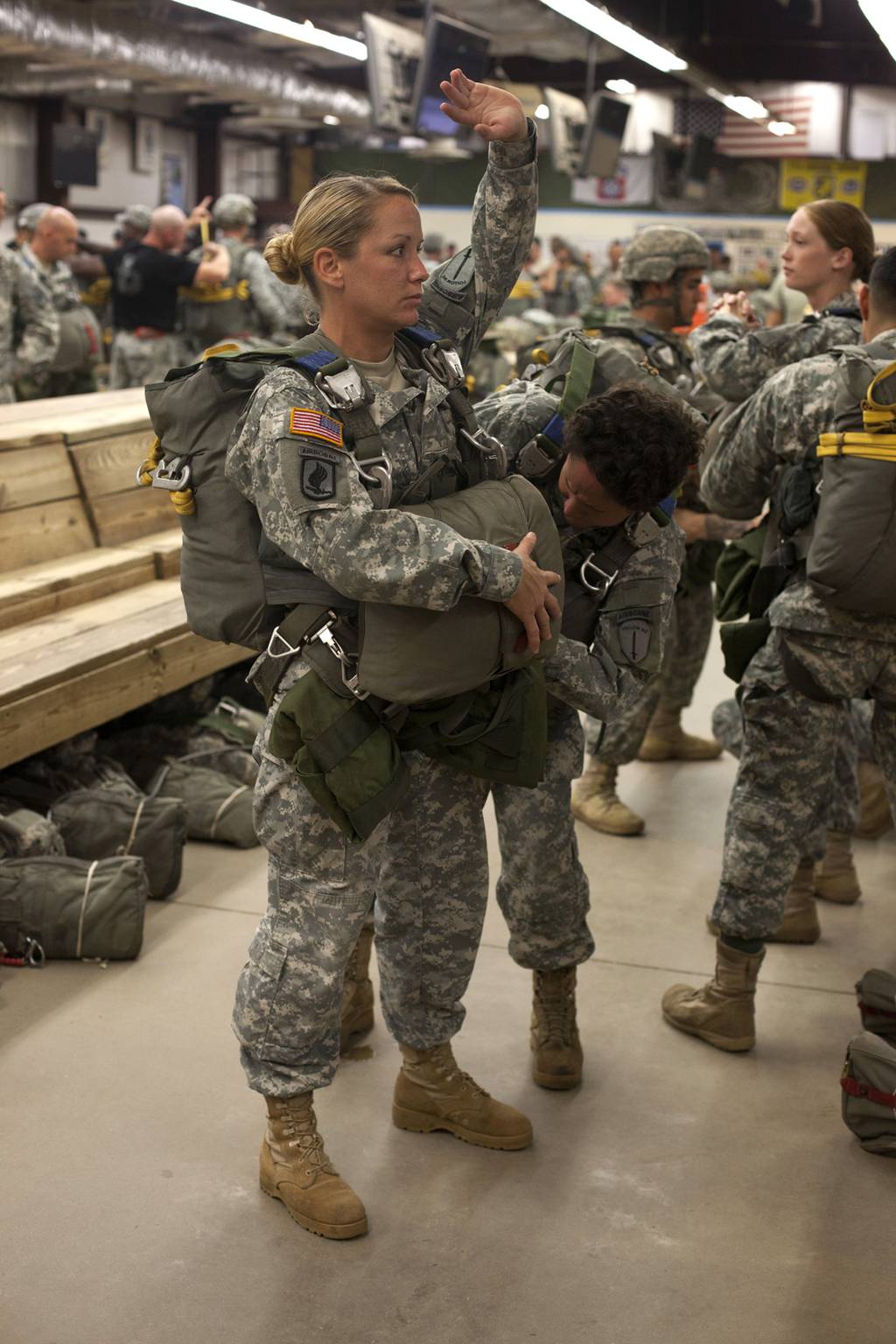The photograph captures a bustling scene of military personnel, likely in a waiting room area such as an airport or a military hangar, preparing for deployment. Prominently in the foreground stands a female soldier with blonde hair tied back in a bun, wearing a full camouflage uniform and tan army boots. She has an American flag patch on her right arm and raises her left hand, seemingly to get someone's attention or respond affirmatively. She carries a knapsack across her chest and has a large backpack on her back. Her expression is one of determination. Near her, a male soldier with an afro leans in, possibly assisting with her gear. To the right, several other soldiers are visible, some wearing helmets and some not, all appearing to ready themselves for departure. A wooden bench to the left supports approximately four or five green duffel bags beneath it, adding to the sense of organized chaos as the troops prepare for their next mission.